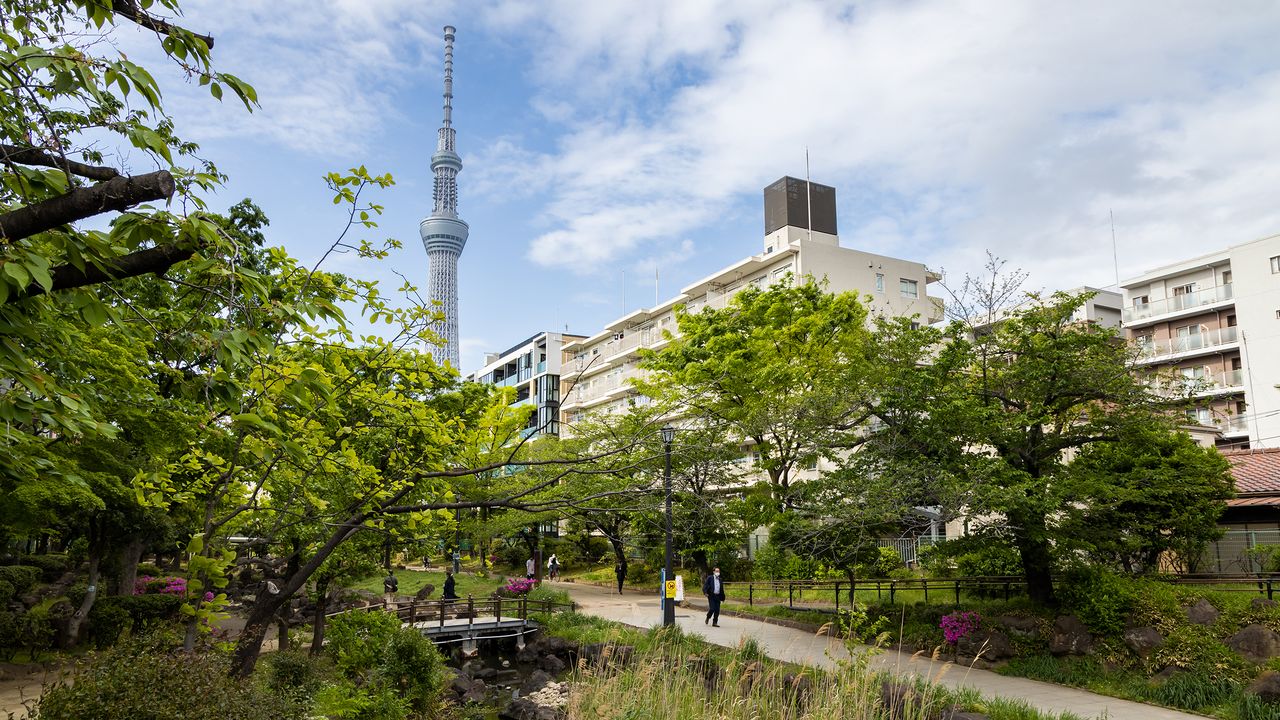This landscape-oriented color photograph captures a serene Asian cityscape, emphasizing its lush greenery and urban elements. Dominating the left edge of the image, a dense cluster of mature, bushy green trees extends with some unusual horizontal branches. A light tan cement path meanders from the lower center to the lower right, intersecting the small city park. Along this path, multiple people walk and bicycle, including a prominent figure in a light blue shirt, blue suit, and white facial mask. In the bottom center, a small footbridge spans a tranquil pool, surrounded by reeds and adding to the park’s charm.

The background reveals two apartment buildings of a whitish hue, one with visible balconies and railings. These buildings are approximately five stories tall and tower over the landscape. In the center-backdrop, a striking tall, needle-like structure, likely made of steel, juts into the light blue sky filled with numerous clouds. The overall scenery, under a sunny sky indicative of spring or early summer, blends verdant natural beauty with urban architecture, creating a vivid snapshot of daily life in an Asian city.